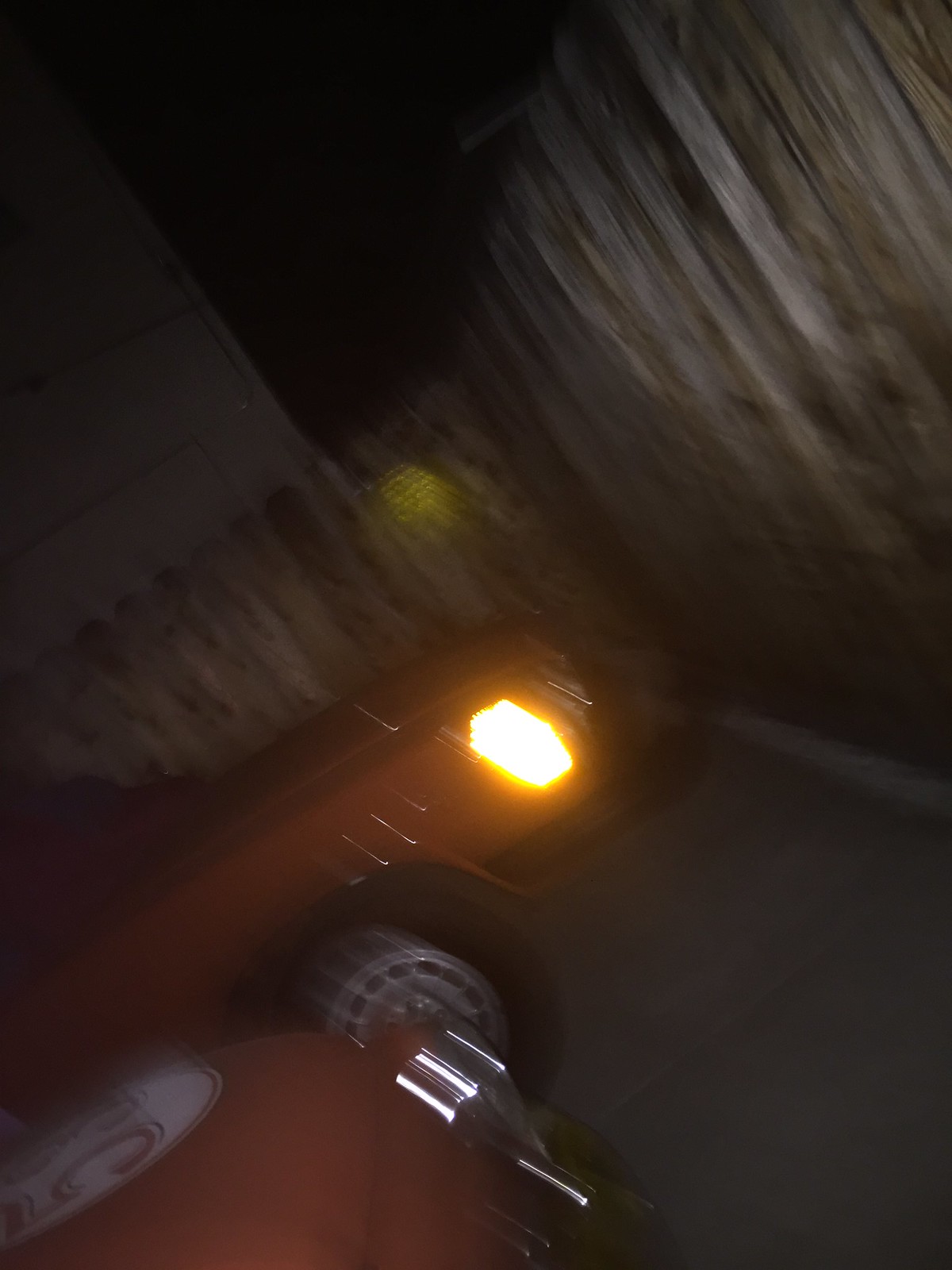This photograph captures a dimly lit night scene featuring a driveway with an orange or red retro-style, boxy car pulling in, its headlights piercing through the darkness. Despite the poor lighting, the car appears to be parked on an asphalt surface and is positioned next to a wooden fence. Adjacent to the car, a vehicle resembling a motorcycle or scooter is visible, distinguished by the number "53" painted in white on its top. The scene also includes a structure, possibly the side of a house or a building, partially visible under the night sky. The image is characterized by significant motion blur, creating streaks of white light and a notable yellow splotch reflecting off the fence from the car's headlight.